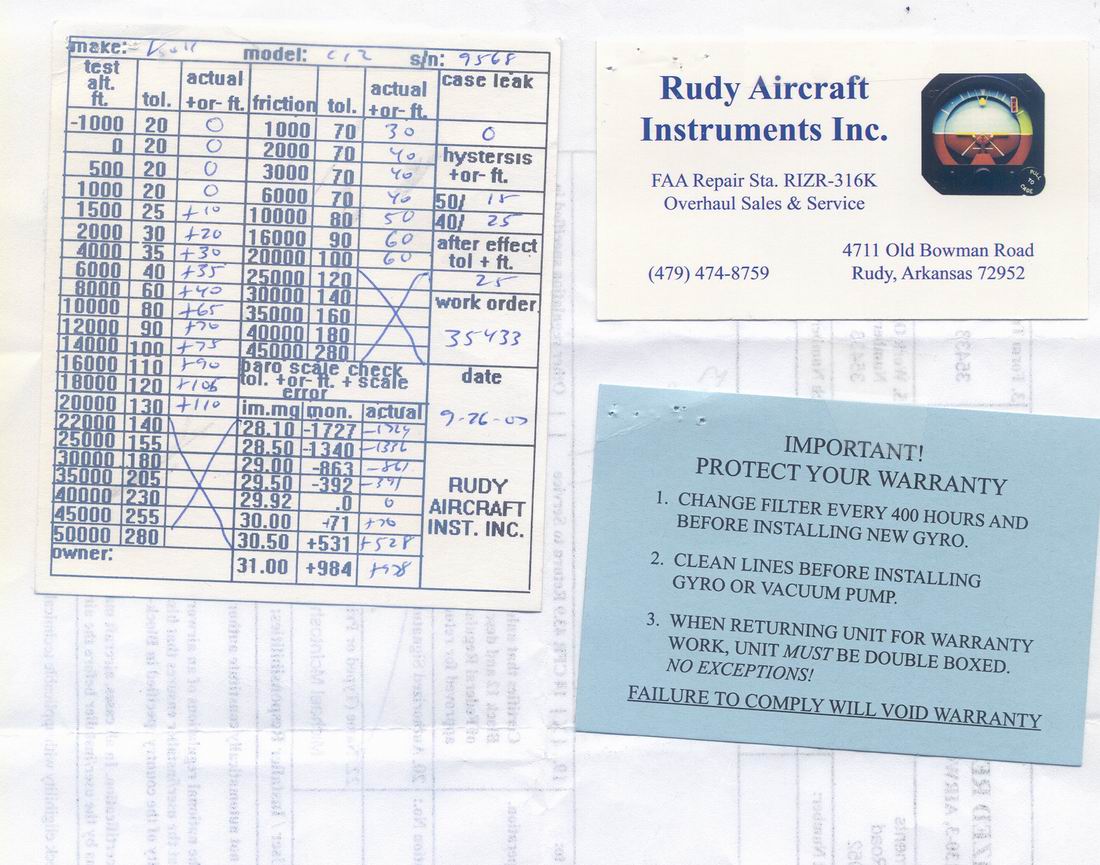The image features a detailed scene consisting of several business and warranty cards laid out over a sheet of paper with visible handwritten data. At the top right, there is a white business card with blue font, which reads "Rudy Aircraft Instruments Incorporated." This card includes details such as "FAA Repair, STA, RIZR-316K, Overhaul Sales and Service," along with the contact number "479-474-8000" and the address "4711 Oldman Road, Rudy, Arkansas, 72952." The top section of this business card includes a square featuring an airplane's leveling instrument. Below this is a blue card with crucial information in black text starting with "Important: Protect your warranty." This blue card lists recommendations for maintenance, such as changing the filter every 400 hours and cleaning lines before installing a new gyro or vacuum pump. In the background, there is a sheet of paper with handwritten columns of numbers and data, possibly from an agreement or work order, listing items like "make, model, serial number," and performance metrics such as "test actual friction actual case leak," followed by "Rudy Aircraft Inc." at the bottom. This paper appears to have been flipped over, revealing some crossed-out entries and a multitude of handwritten annotations.